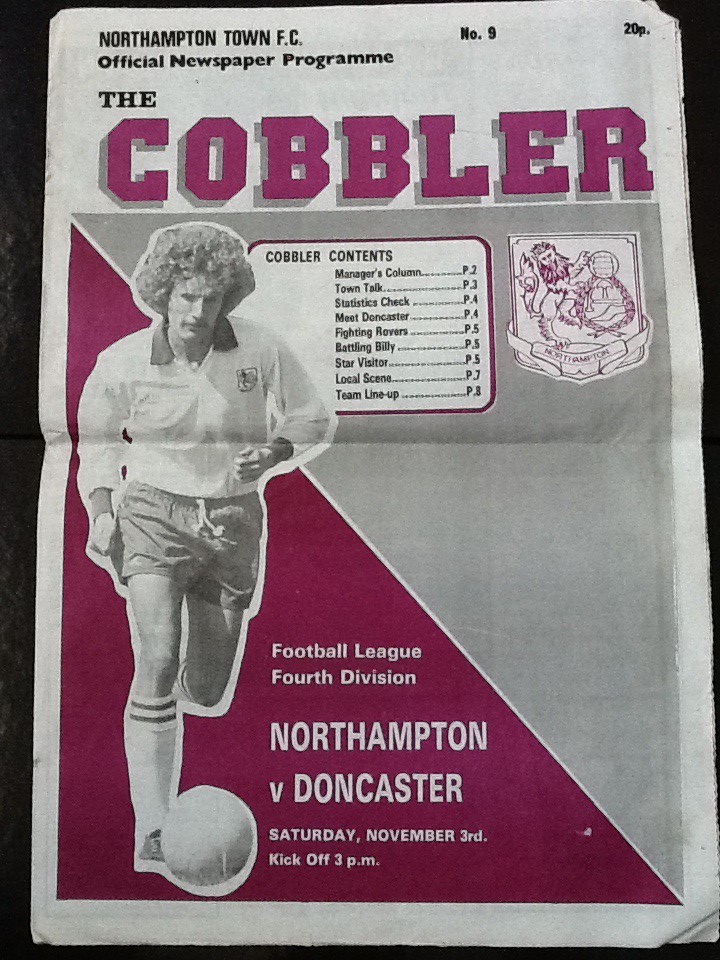The image is a scanned cover of an old, worn-out soccer program, identified as the Northampton Town FC Official Newspaper Program titled "The Cobbler." The edges are visibly creased and bent, indicating it has been folded in half from top to bottom. At the top left, the program prominently displays "Northampton Town FC Official Newspaper Program, The Cobbler" in purple text on a white background. 

Beneath this header, the contents are listed under the section titled "Cobbler Contents," detailing various sections such as the Manager's Column, Town Talk, along with team statistics and discussions on the local scene and visiting teams. The cover is artistically divided with a diagonal line, creating two halves: the left half in purple and the right in gray. In the bottom left, a black and white photo of a soccer player from the 1960s or 70s is captured mid-action, about to kick a ball. 

In the top right corner, the price of "20 pence" is printed, and further down below the contents list, there's a match announcement for the Football League Fourth Division game between Northampton and Doncaster, scheduled for Saturday, November 3rd, with a kickoff at 3 p.m. An insignia featuring a lion appears on the far right of the cover, completing the nostalgic and detailed design of this vintage soccer program.